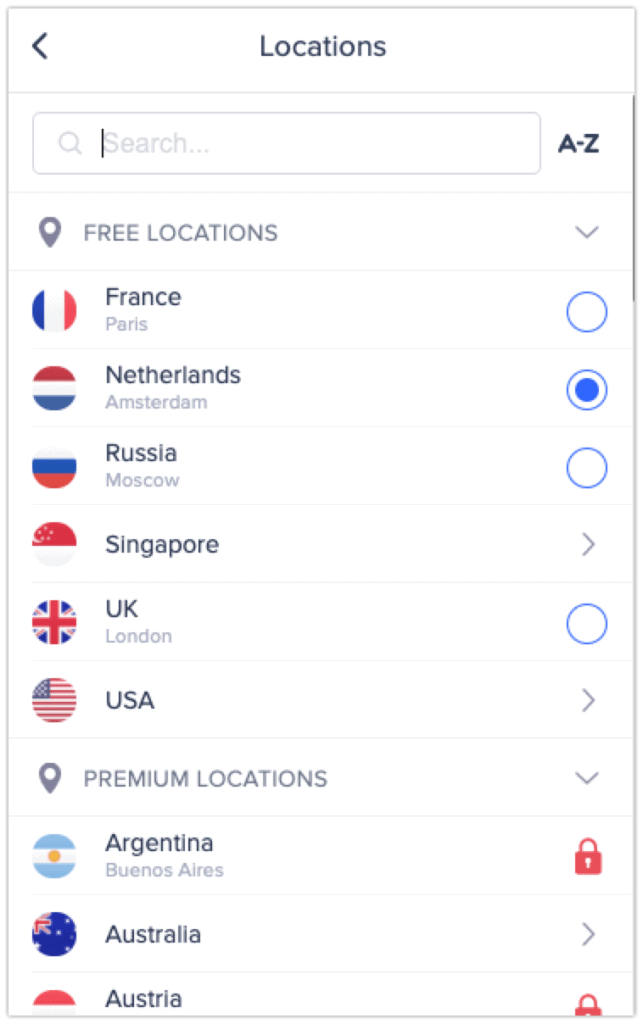The image is titled "Locations" at the very top of the screen against a completely white background. Directly below the title, there is a small search data window with the letters A to Z on the far edge for alphabetical sorting. The search window is followed by a list where lines of text start with the grayed out heading "Free Locations."

In the list of international locations, there are round flag symbols on the left side representing different countries, and on the far right of each row, there is a round selection circle. The list begins with France and descends in alphabetical order to the Netherlands, Russia, Singapore, UK, and USA. The Netherlands is indicated as being selected by a right-hand round circle that features a dark blue dot in its center.

Further down, there is a subsection titled "Premium Locations," which displays three countries: Argentina, Australia, and Austria. Next to each country's name, there are smaller text identifiers, such as "Buenos Aires" for Argentina. On the far right side of each premium row, a red locked icon signifies that these locations are not freely accessible.